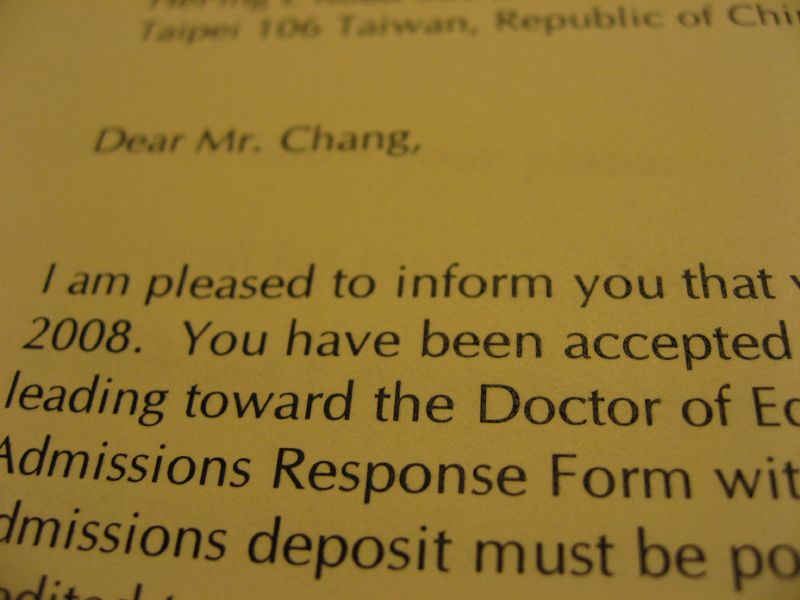The image is a zoomed-in photograph of a yellowed, beige sheet of paper that appears extremely well-preserved, showing no signs of wrinkling or weathering. The text, written in black, is partially visible due to the diagonal orientation of the paper in the image. At the top, the text reads "Taipei 106, Taiwan, Republic of China," followed by "Dear Mr. Chang." The letter mentions a date from 2008 and indicates Mr. Chang's acceptance into a program related to a Doctor of Education. Specific details about the admissions response form and deposit requirements are partially cut off, making the full content difficult to discern. Despite the aged appearance of the paper, the content suggests it is more recent, originating from 2008. This letter is addressed to Mr. Chang and seems to be associated with an academic acceptance in Taipei.